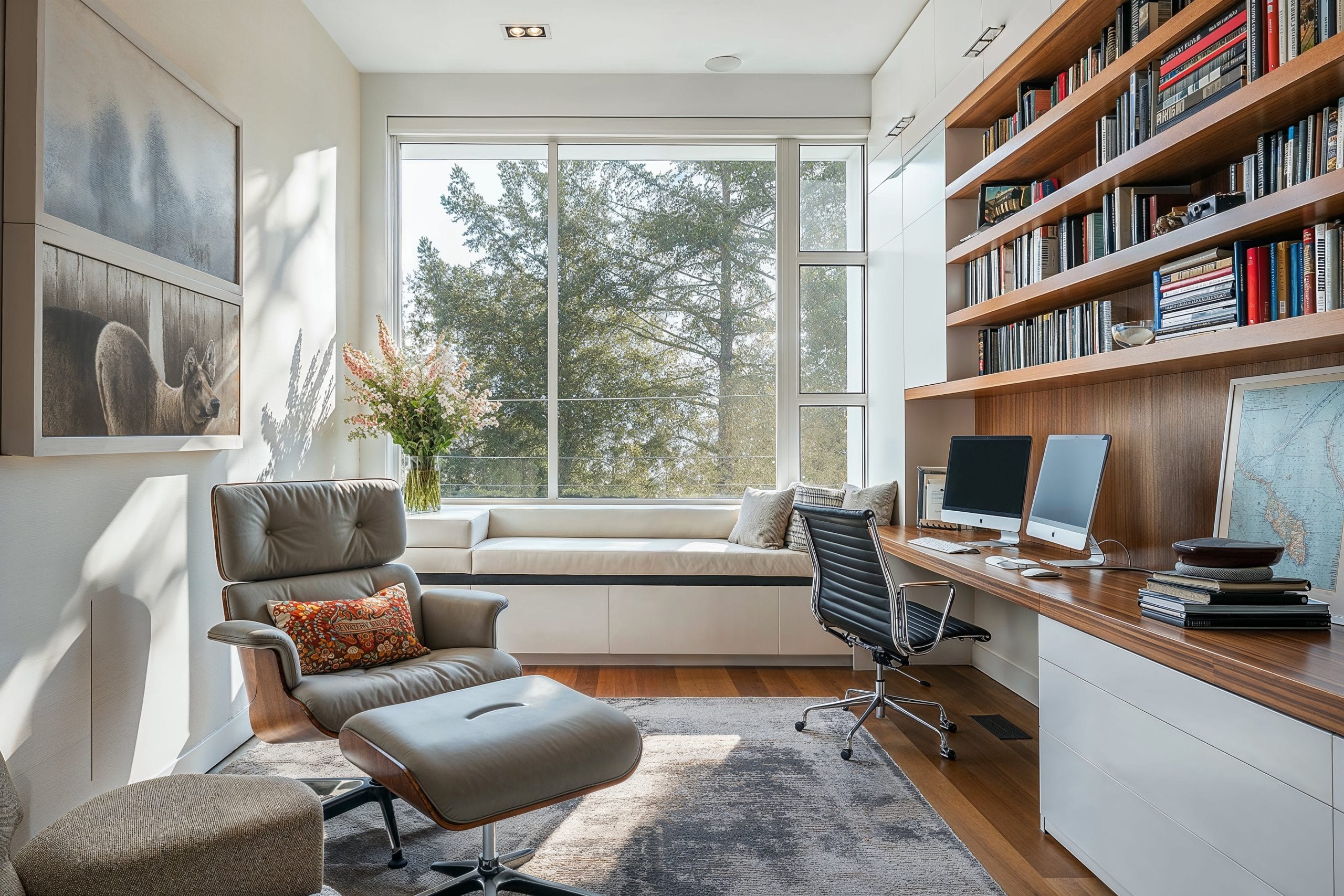This is a detailed photo of a modern home office, captured from the doorway. The focal point of the room is a large picture window at the very back, through which tall trees are visible, indicating a wooded area outside. The sunlight pours through the window, casting vivid shadows on the left wall. Directly beneath the window, there's a light tan or cream-colored sofa with a flower pot placed on its arm, which serves as a window sill or a seating area.

On the left wall, there's a sizable framed picture featuring an upper and lower panel, depicting trees and, potentially, an animal which could either be a dog or a deer. Below this picture, there's a modern light brown chair with arms and an extended footrest.

The right-hand side of the room features a built-in desk and bookcase arrangement. The upper section consists of four horizontally arranged shelves filled with books. The lower section is a long desk surface with two Mac computer screens, various office items, and an office chair tucked underneath. Built into the desk are several filing cabinets.

The flooring is wooden with a large gray rug placed centrally. The room is bathed in natural light, creating a bright and peaceful ambiance with a color palette of wood, gray, and white tones. The overall atmosphere reflects a serene and well-organized working space.